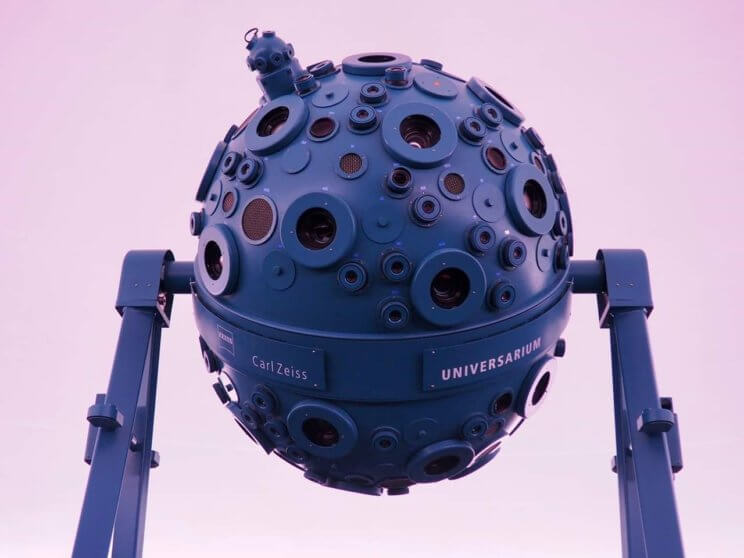The image depicts a large, spherical projector used in a planetarium to project stars and celestial images onto a dome. The orb, crafted from a deep blue material, is adorned with slightly raised crater-like circles, each housing multiple lenses, cameras, and projectors. The sphere is prominently branded with the names "Carl Zeiss" on its left side and "Universarium" on its right, signifying its high-quality lens design and specific model type. The projector is suspended in mid-air by two blue, A-frame metal arms, ensuring its stability and allowing it to pivot freely to accurately project images across the dome. The backdrop of the image is a light, pinkish-purple hue, enhancing the contrast and detail of the blue orb and its support structure.